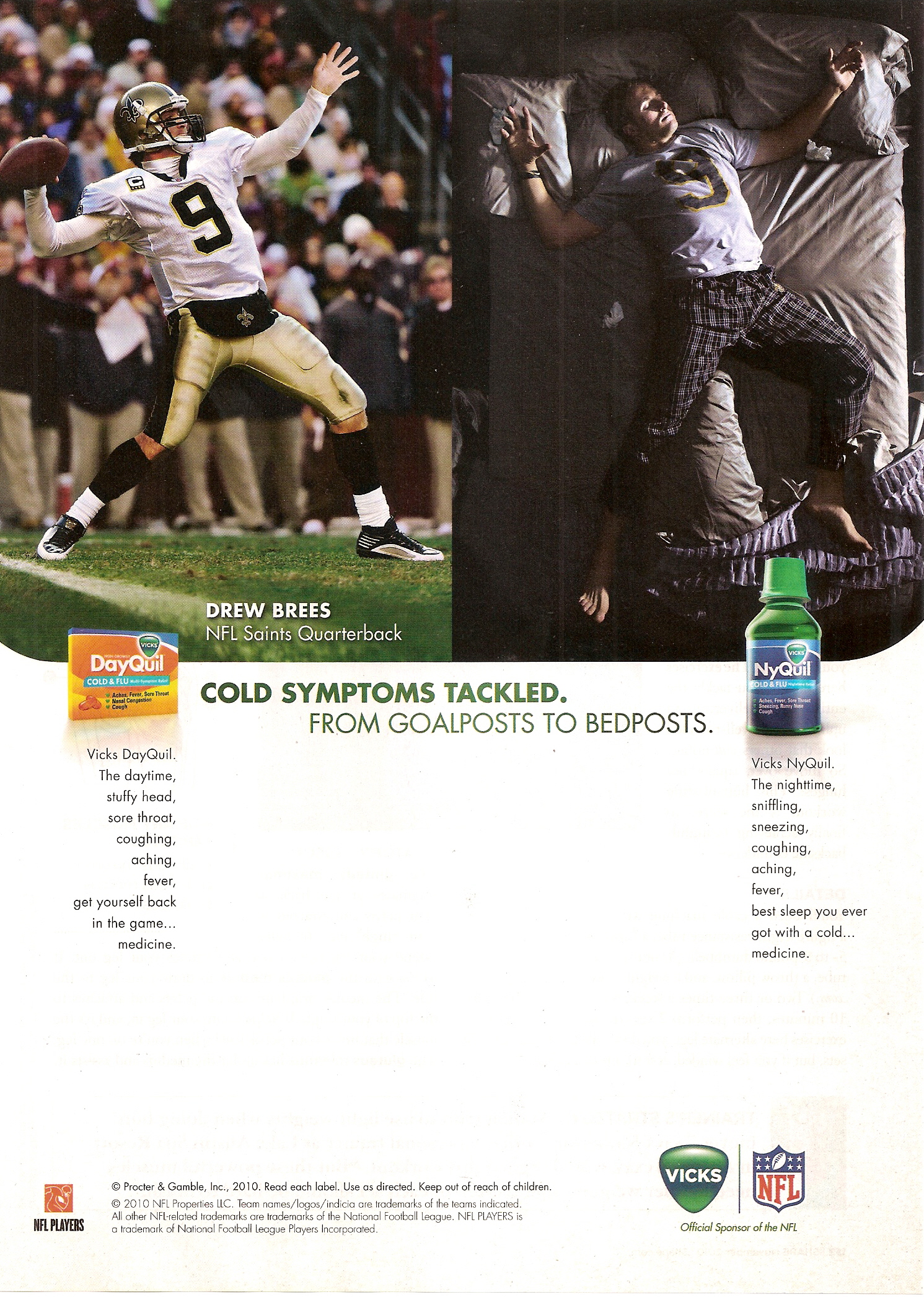This advertisement for Vicks prominently features NFL quarterback Drew Brees in a dual scene. On the left, Brees is depicted mid-throw during a football game, wearing his white jersey with a large black number 9 and gold pants, against a backdrop of fans in the stadium. On the right, Brees is shown lying in bed, dressed in pajamas that mimic his football attire, in the same throwing pose, with a blanket kicked off at the bottom of the bed. Below these images is the tagline, “Cold symptoms tackled from goal posts to bed posts.” The left side of the ad displays a box of DayQuil tablets, while the right showcases a small bottle of NyQuil syrup. At the bottom, logos for the NFL Players Association, Vicks, and the NFL underscore the message, with additional text emphasizing Vicks as the “official sponsor of the NFL” and promoting DayQuil for daytime relief and NyQuil for nighttime symptoms, encouraging cold sufferers to "get back in the game."